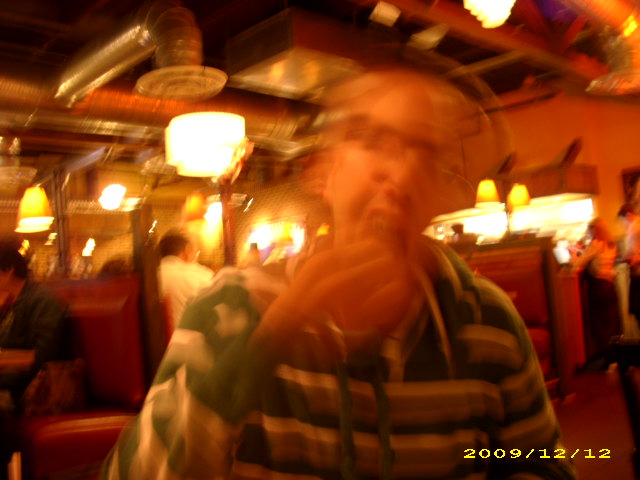A blurry photograph taken inside a restaurant captures a dynamic scene. In the background, there are booths filled with people, featuring distinctive red leather seats. In the foreground, a male figure is the main subject, but his rapid movements and the low lighting make his head and arm appear very blurred. He seems to be in the middle of eating, with his mouth open and one hand holding food up to his mouth. The man has short hair, appears to be white, and is wearing a pullover hoodie with dark green, white, and gray horizontal stripes. A date stamp on the bottom right corner of the image shows "2009-12-12."